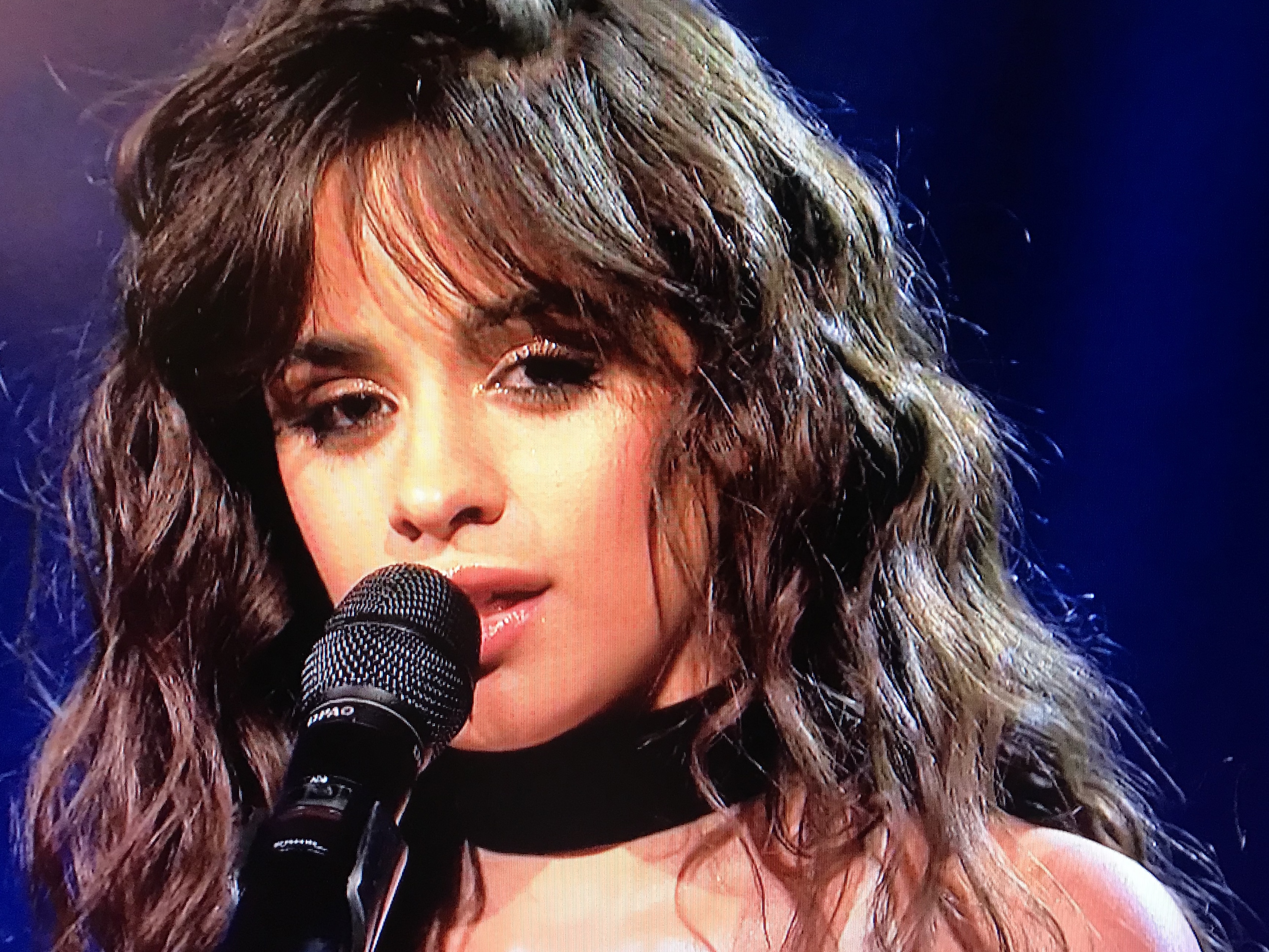In this photograph, a famous singer, possibly Aria Grande or Camila Cabello, is captured mid-performance. The shot is a close-up, zoomed in on her face and cutting off at her shoulders. She has long, wavy black hair with bangs falling softly over her forehead and her shiny, natural-looking lip gloss highlights her lips as she sings into the microphone, which is positioned right at her lips. She wears a distinctive black choker necklace, possibly velvet, complementing the dark hues of her attire. The background features varying shades of blue, illuminated by stage lighting that casts a glow on her left shoulder and hair, enhancing the vibrant atmosphere of the performance.